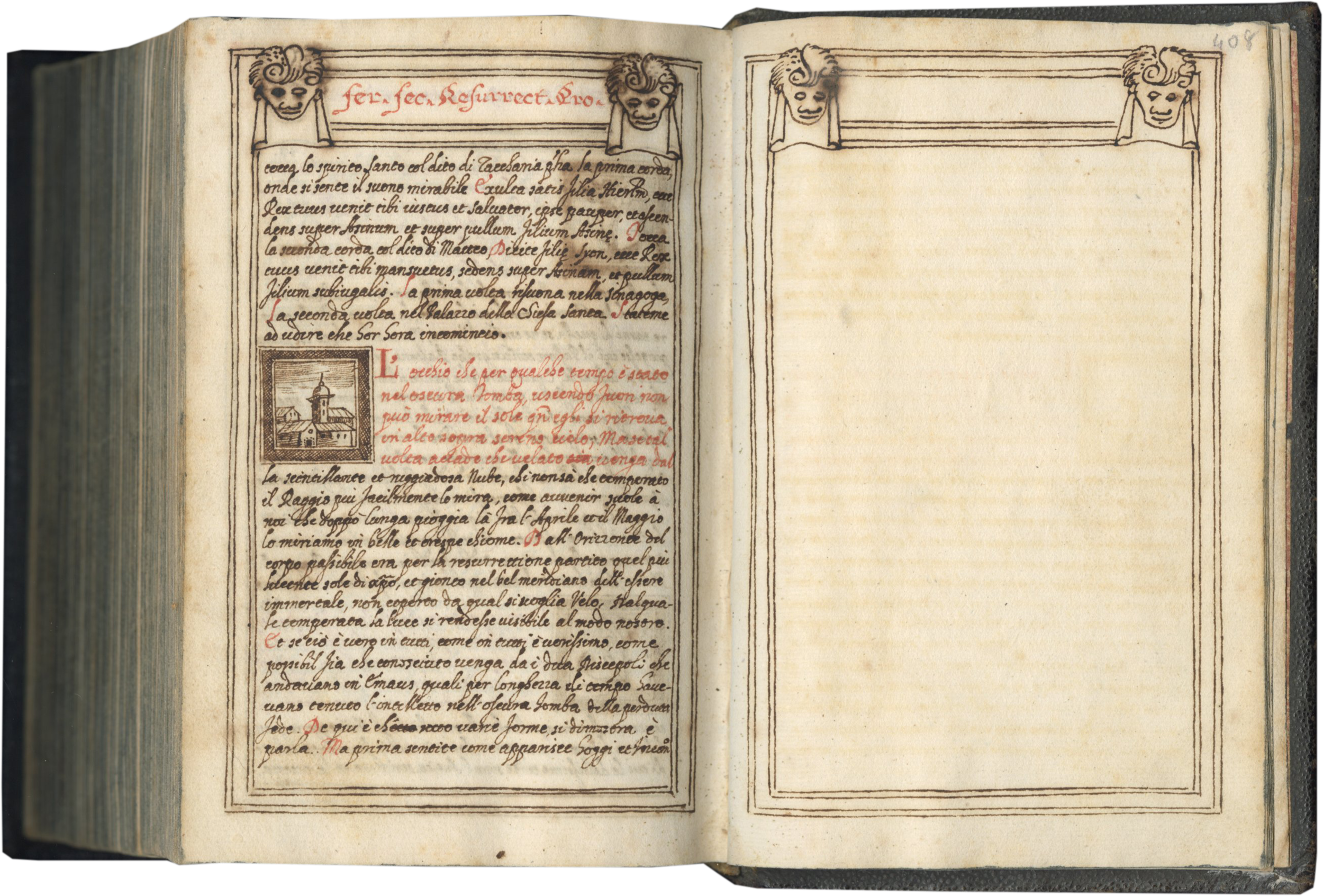The image portrays a very old and large book, open to show its pages. The book, which appears to have a black outer cover, has yellowed, cream-colored pages indicative of its age. The left page contains intricate red and black text in very small lettering, possibly in Latin, with the text formatted in such a way that the header and the initial letters of the paragraphs are in red. A paragraph written in black cursive follows the header. Midway down the page, there is an illustration depicting what appears to be medieval buildings, possibly a small church or a tower, accompanied by descriptive text in red. Below this, another paragraph in black cursive fills the remainder of the page.

At the top of each page are ornate decorations featuring cherubs or faces with a banner between them, intended for titling. The right page is entirely blank, except for these decorative elements at the top. The scene is set against a simple white background, which draws focus solely to the book and its detailed contents. The pages are heavily worn, further emphasizing the book’s ancient character.